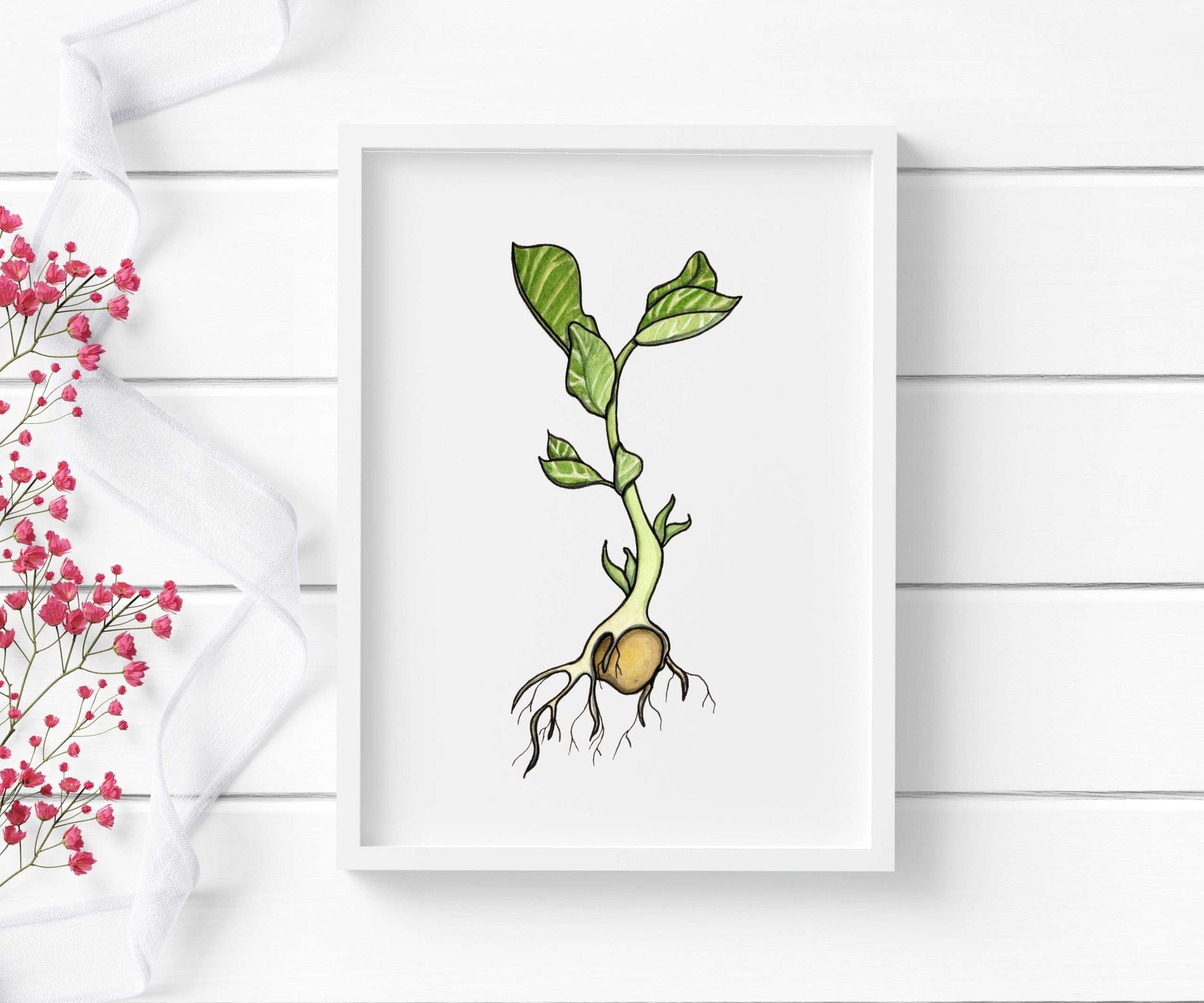The image depicts a detailed drawing of a green-rooted plant, likely an onion, showcasing a robust root structure at the bottom. Green leaves extend upwards from a prominent stem, which captures the natural essence of the plant. This artwork appears to be rendered with markers, contributing to its vivid portrayal. The drawing is set inside a white picture frame, blending seamlessly into the white background. This white background features subtle indented lines, reminiscent of wooden planks, suggesting a textured surface, possibly a white table or wall. To the left of the drawing, there are delicate pink flowers on green twigs, captured partially, adding a touch of color and contrast. A white cloth spirals gracefully across this section, enhancing the overall aesthetic and compositional balance of the image.